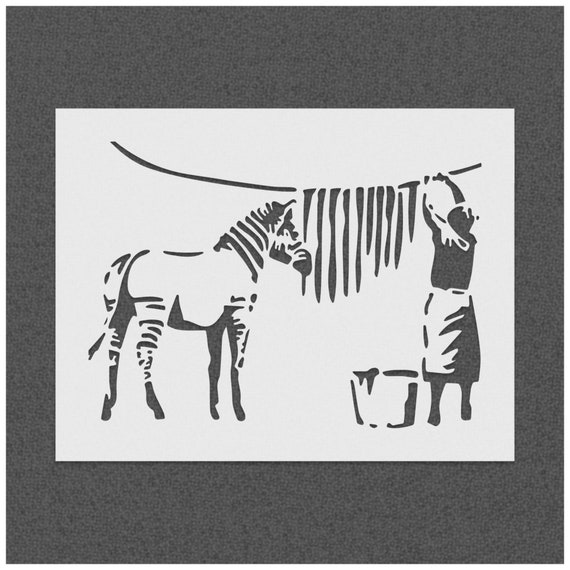This illustration, set against a very pale blue background and framed by a textured dark gray border, features a whimsical yet evocative scene in stark black-and-white silhouettes. To the right, a woman stands with her back facing the viewer, reaching up to hang laundry on a clothesline that stretches across the image. She's dressed in a long-sleeve top and skirt, discernible by their contrasting shades of black and white. Below her, to the left, rests a wash bucket. The clothesline holds several black stripes, hanging vertically, which intriguingly appear to be the missing stripes of the zebra depicted to the left of the scene. The zebra, characterized by its distinct head and leg markings, gazes towards the woman. Its body is predominantly white, accentuating the humorous implication that its stripes are being washed and hung to dry. This surrealistic touch is captured in an abstract yet easily interpretable manner, creating a visually engaging and thought-provoking image.